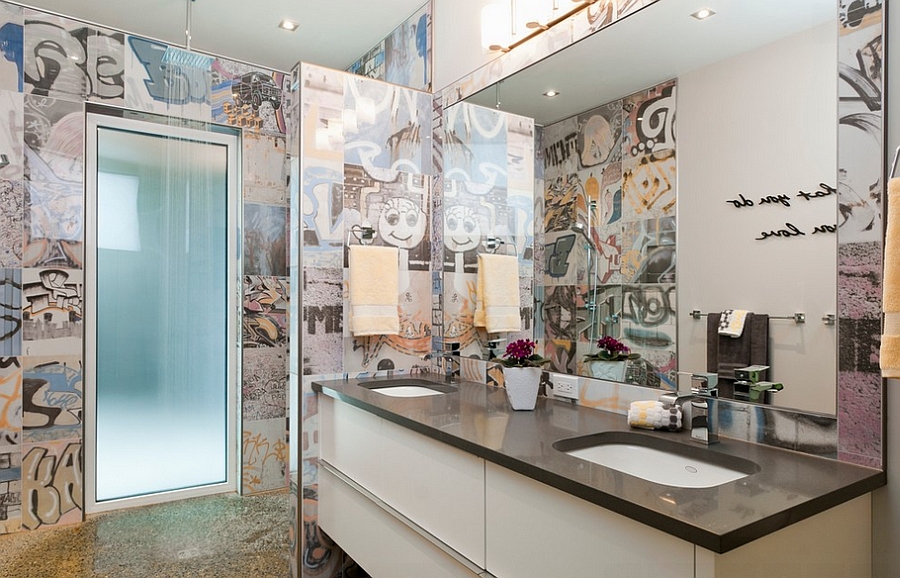This indoor color photograph captures a spacious, modern bathroom with a dual vanity setup. The vanity features a sleek black countertop with two white sinks and polished nickel faucets, characterized by their rectilinear, blocky design. The countertop is contrasted by a floating ivory-colored cabinet with white drawers on the sides. Above the vanity, a large mirror spans the width of the room, reflecting the vivid and eclectic graffiti-inspired wallpaper that covers the walls. This wallpaper consists of abstract and cartoon-like designs in muted tones of beige, gray, blue, and yellow, creating a visually busy atmosphere.

To the left of the vanity is a frosted glass shower door, adding to the room's contemporary aesthetic. A bright yellow towel hangs on the wall near the leftmost sink, adding a pop of color to the scene. Between the two sinks, a white vase with a red flower adds a touch of elegance. The bathroom also features subtle ceiling lights that illuminate the space, highlighting the colorful and intricate wall art. Additionally, a reflection in the mirror hints at some cursive writing on the opposite wall, though it's not entirely legible. The overall design is an amalgamation of modern and abstract elements, creating a distinctive yet busy vibe in the bathroom.